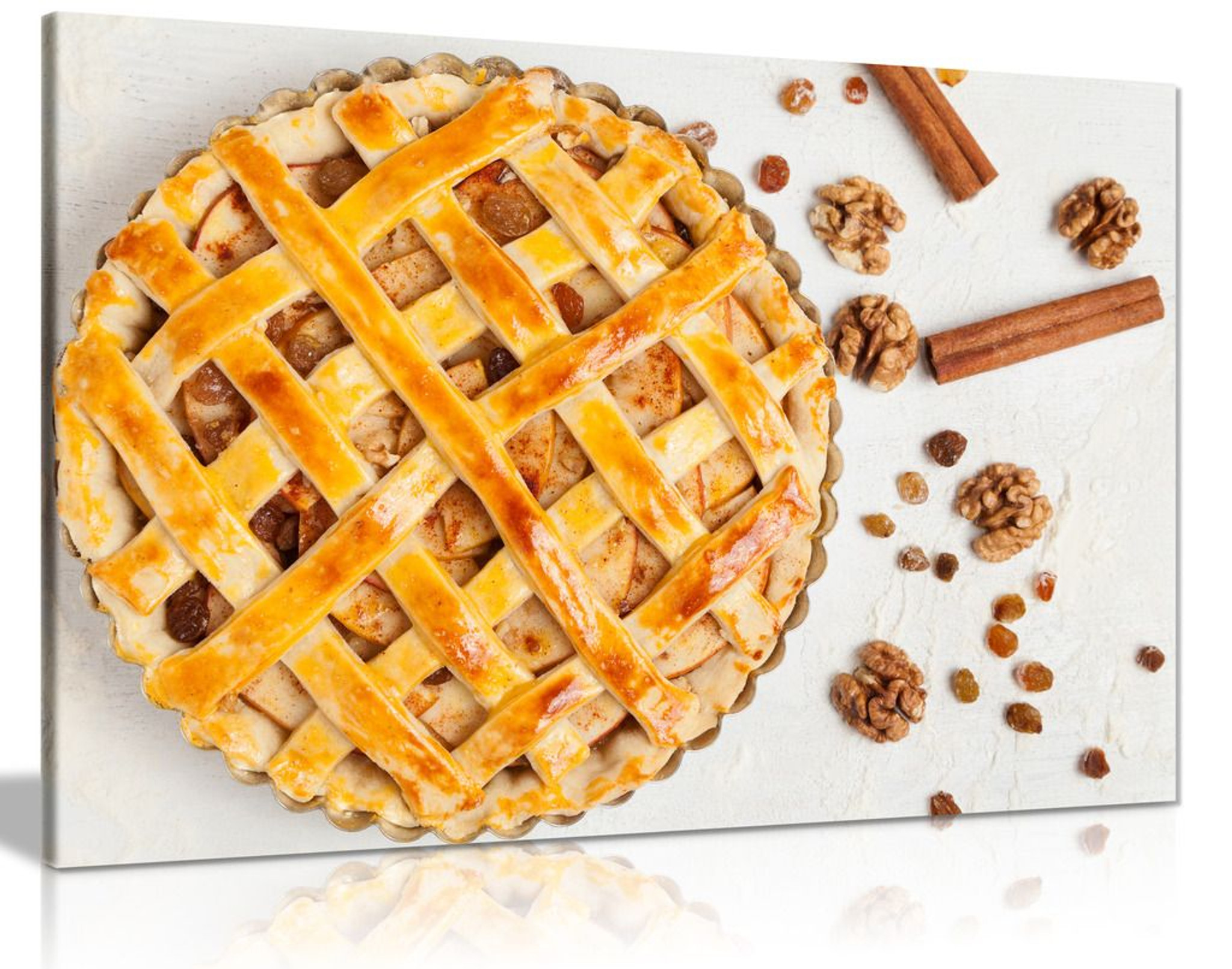This is an elevated photo showcasing a beautifully glazed, lattice-topped apple pie, captured against a stylish countertop or poster board. The photograph prominently displays the pie's intricately woven crust, created by overlapping strips of dough that have been brushed with egg wash for a shiny, golden-brown finish. The upper right portion of the image is adorned with assorted nuts, likely walnuts or pecans, and cinnamon sticks, adding a rustic charm. The backdrop features a collection of these elements scattered around, enhancing the overall visual appeal and emphasizing the pie's delicious ingredients.